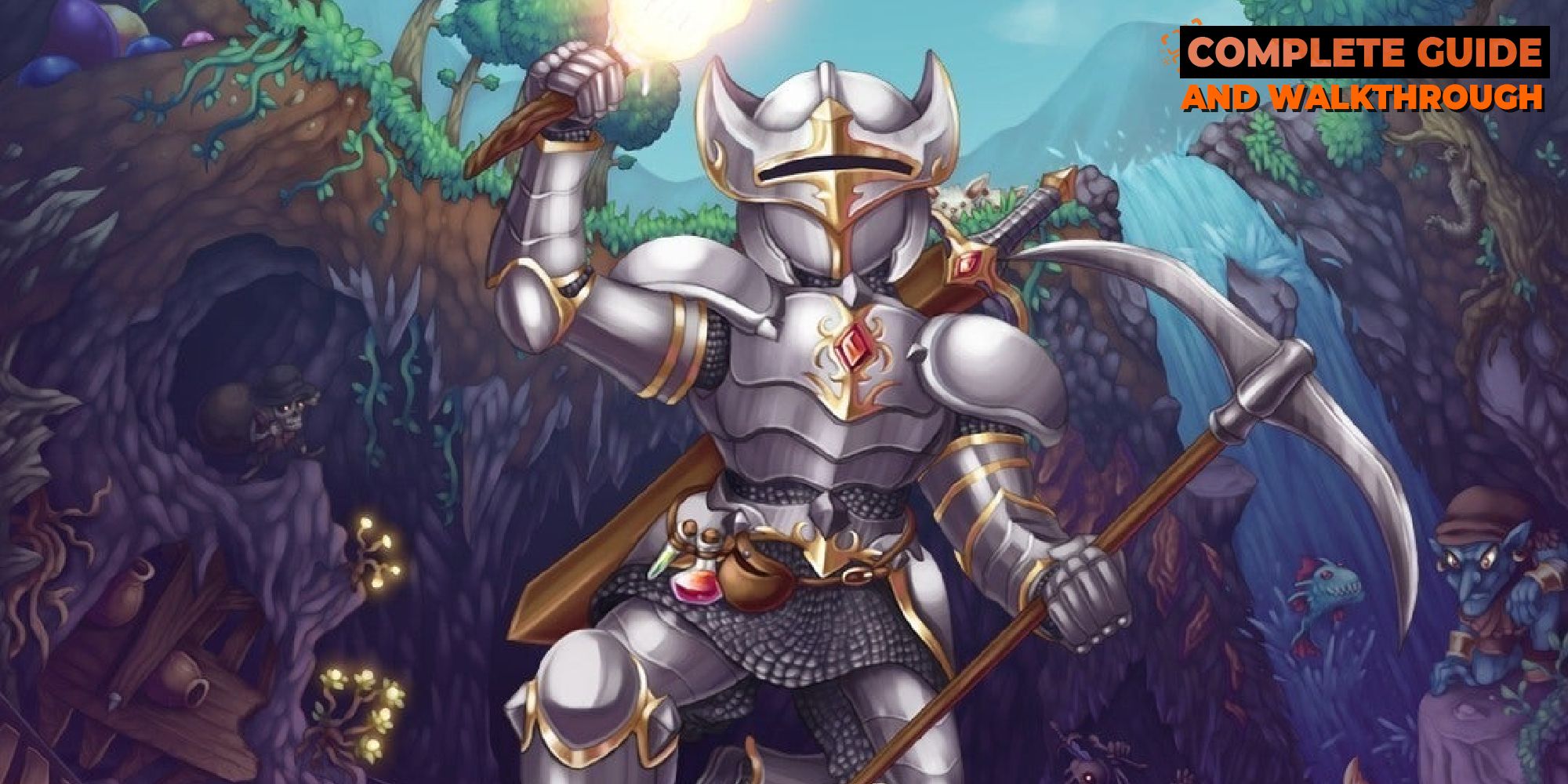The image appears to be a vibrant, computer-generated digital artwork from a game, indicated by a "Complete Guide and Walkthrough" sign in the top right corner, written in light yellow and orange letters against a black rectangle background. The scene is set outdoors, possibly in a rainforest, with lush trees at the top, a bright sun, a cascading waterfall on the right, and rocky cliffs. On the left side, there's a cave opening with flowers, wooden areas, a fence, and pots scattered around. The focal point is a knight standing in the middle, clad in silver and gold-plated armor with chainmail, a helmet, and completely obscured skin. The knight carries a double-sided silver axe with a brown handle in their left hand and a wooden stake or dagger in their right hand, which could be a light source. Additionally, the knight has a sword sheathed on their back and various items like potions and a ruby embedded in the chest armor. Around the knight, there's a sense of foreboding with lurking creatures, including a small blue, gremlin-like creature with clothing and a hat in the bottom right, and possibly a fish or skeletal figure in the background, suggesting the knight is venturing into a dark, eerie, and forbidden area.